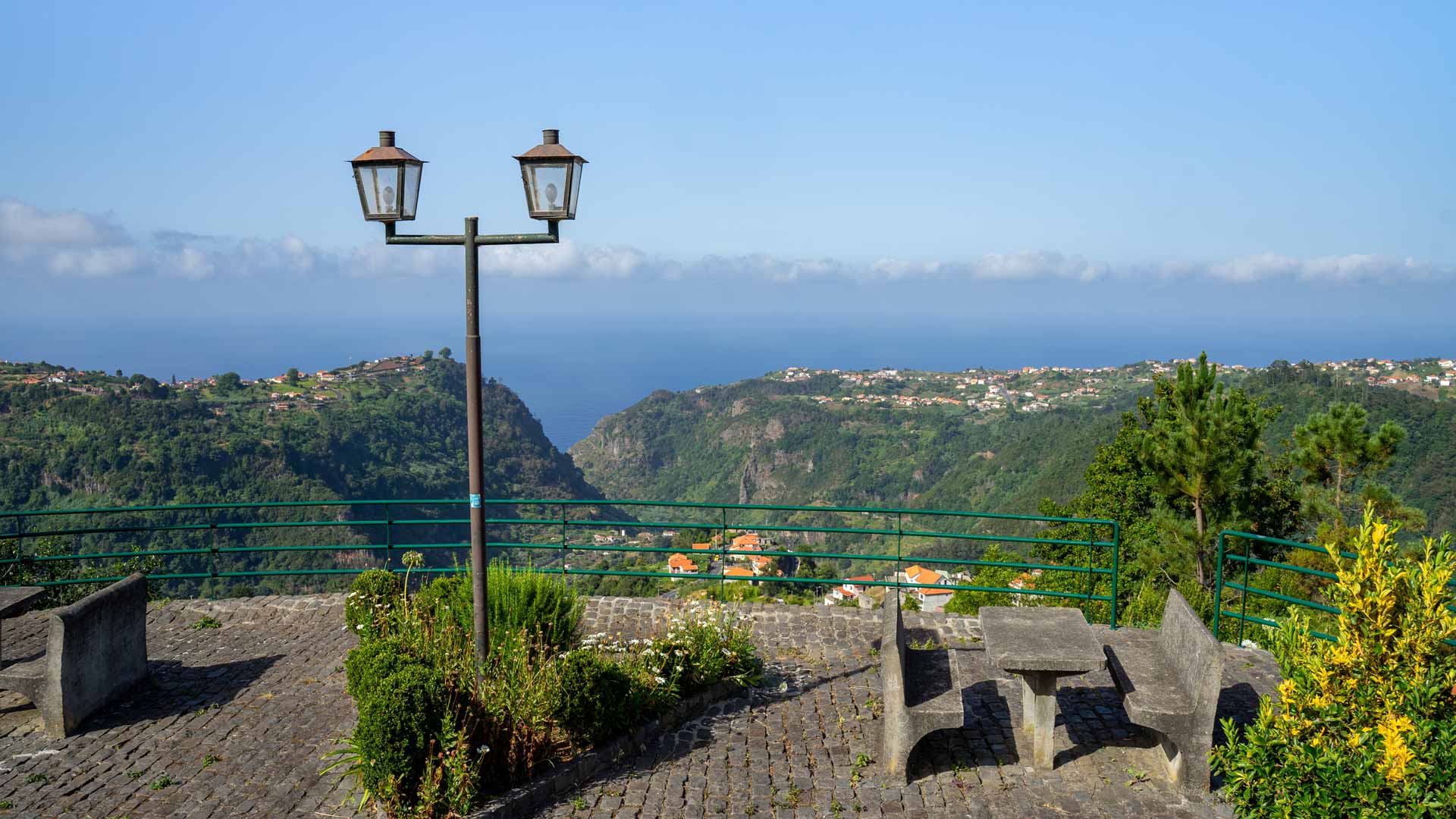This high-resolution photograph captures an overlook from a concrete ledge adorned with cobblestones. The vantage point offers a sweeping view of a valley nestled between hills and mountains, culminating in a bright blue sky filled with scattered clouds. In the distance, white homes crowned with orange rooftops dot the landscape, possibly near a body of water like the sea or a river. Close to the camera on the right, a prominent green tree adds to the verdant scenery. The ledge is bordered by a green guardrail that runs from left to right, ensuring safety while admiring the view.

On the left side of the ledge, a green tree with hints of yellow stands nearby a concrete bench angled upwards. Adjacent to this bench is another concrete bench facing it, with a table set between them. Further left, a black lamppost rises from the concrete, bifurcating into two arms each topped with a clear, white globe light, capped in black. Greenery surrounds the base of the lamppost, enhancing the natural beauty of the setting. The overall scene is a harmonious blend of gray, green, blue, and splashes of natural hues, creating a picturesque and peaceful overlook.